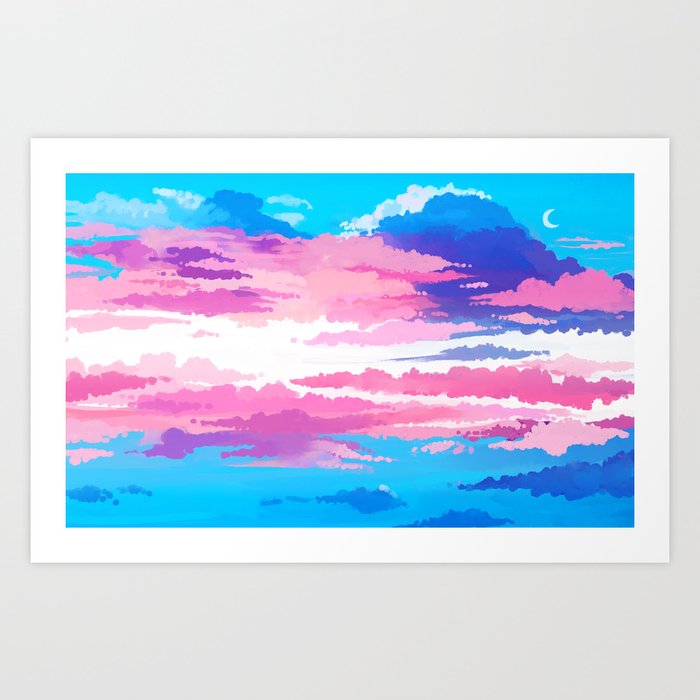On a light gray wall hangs a large horizontal rectangular art print, featuring a serene and colorful sky. The picture has a prominent thick white border, enhancing its visual appeal. The sky illustration transitions from light blue at the top to darker blue hues at the bottom. Dominating the upper right corner is a delicate white crescent moon, its tips pointing to the right. This sky scene is populated with a diverse array of clouds, primarily in shades of blue, pink, and purple, blending harmoniously.

In the upper section, there are medium and dark blue clouds mingled with white ones. Especially notable are two main clouds: a medium blue cloud on the left and a darker blue cloud on the right, with a white cloud interplaying with the darker blue on the right side. A striking white horizontal stripe cuts across the middle of the image, bordered by a mix of cloud types. Towards the middle section, a large area showcases overlapping clouds in dark blue, pink, and white, transitioning into darker pink and purplish shades below. The lower portion is a soft continuation of this gradient, marked by light blue and dark blue clouds completing this vivid atmospheric artwork.